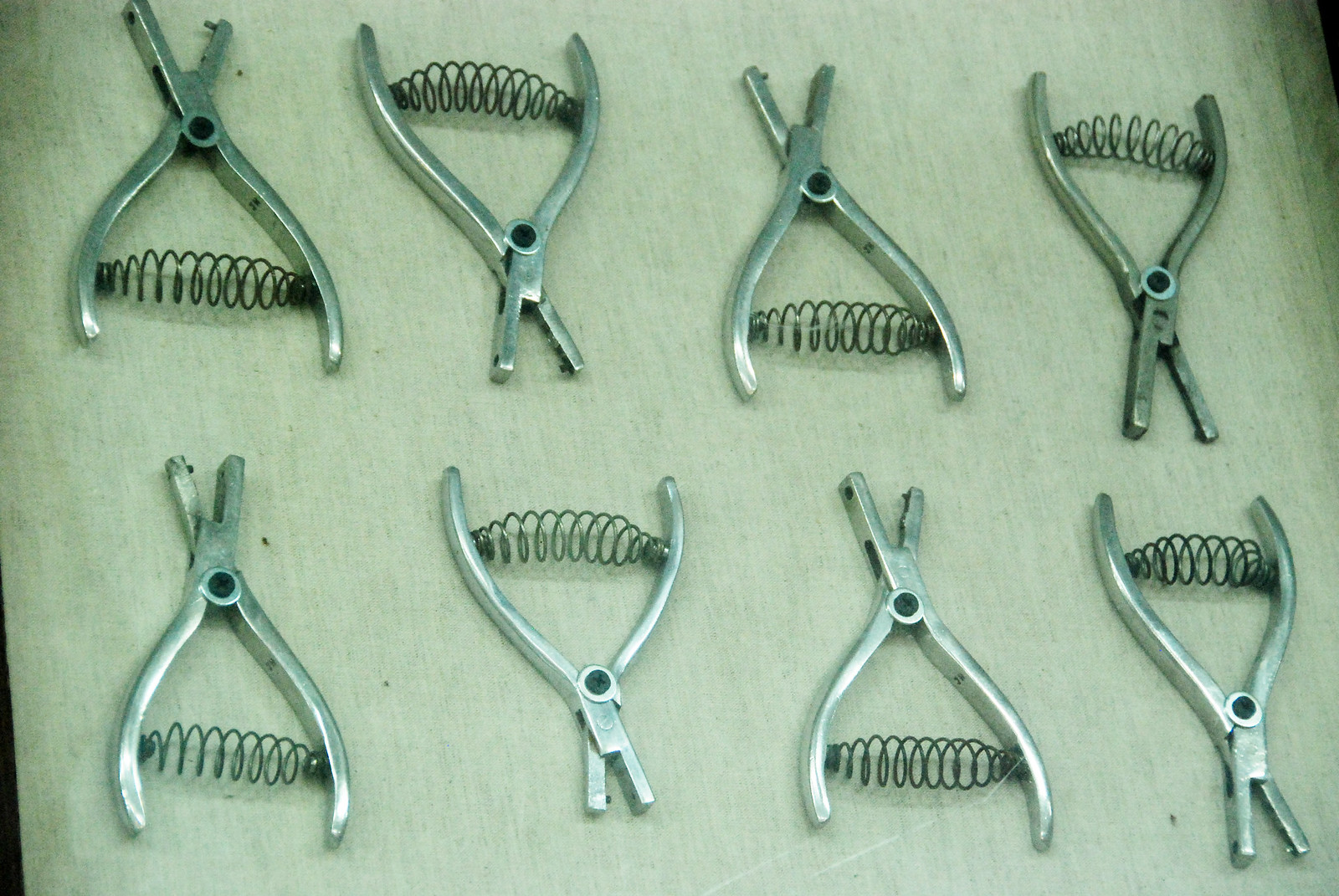In this rectangular image, we're looking at a photograph taken from above that depicts eight identical stainless steel grip tools resembling small pliers. These tools are neatly arranged in two rows of four, with their orientations alternating—one facing up, the next down, and so on. They are positioned on a light tan wood surface. Each tool features a rounded rectangular handle with a black, accordion-like spring running horizontally across the left and right sides of the arms, which widens at the center to facilitate opening and closing the gripping end. The background has a muted greenish-gray tone, and the overall setup suggests they could be specialized tools for handling animals or detailed grip work.